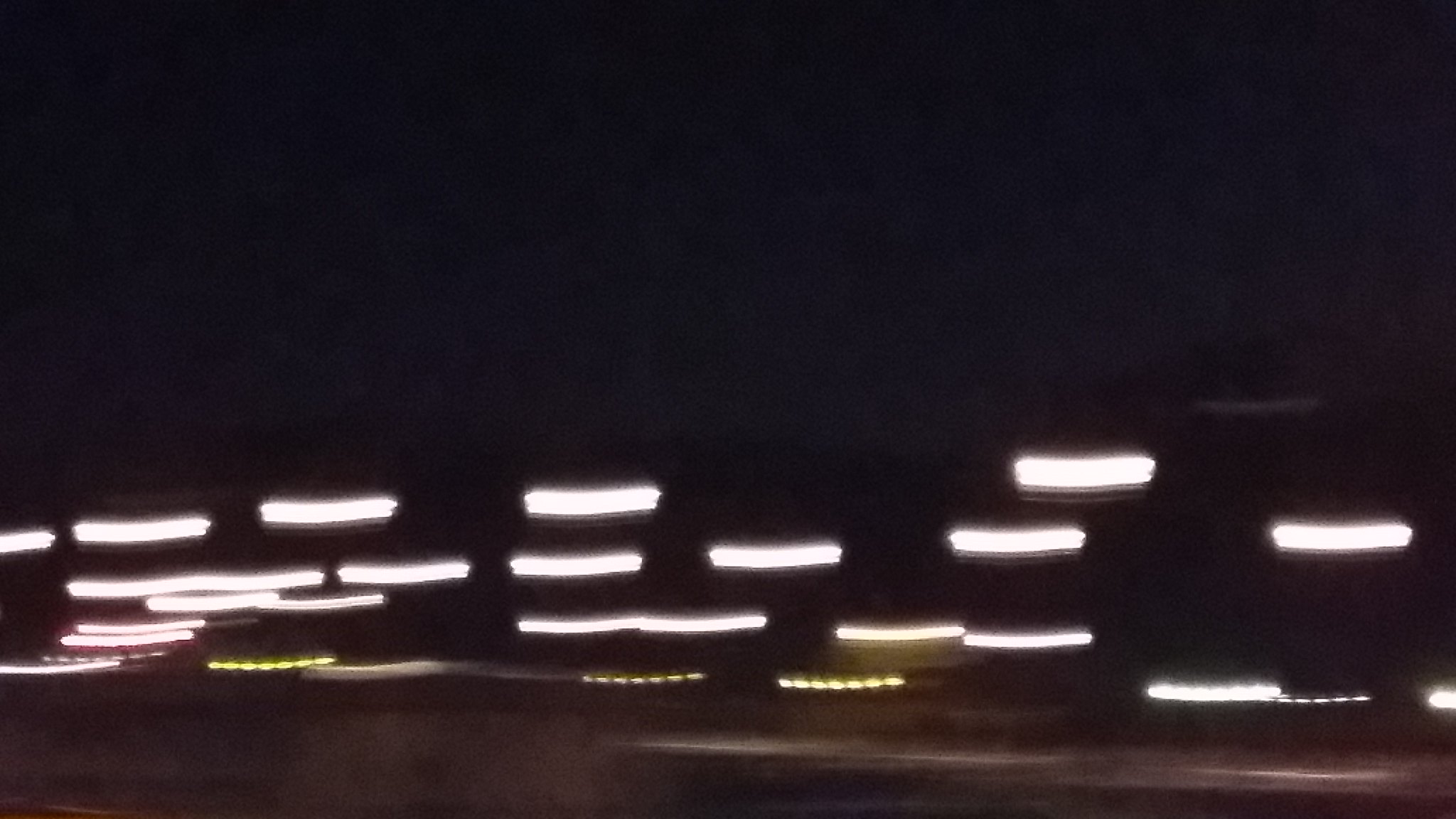A blurry photograph showcasing an array of unidentified lights against a predominantly black background. The upper section of the image is enveloped in darkness, gradually lightening towards the bottom. The lights are organized in four irregular, horizontal rows, with larger lights at the top and a narrow, tightly-packed row at the bottom. The exact nature of these lights remains indeterminate – they could be neon, industrial, or another type. The overall scene gives the impression of peering at a possibly illuminated structure or area shrouded in obscurity.